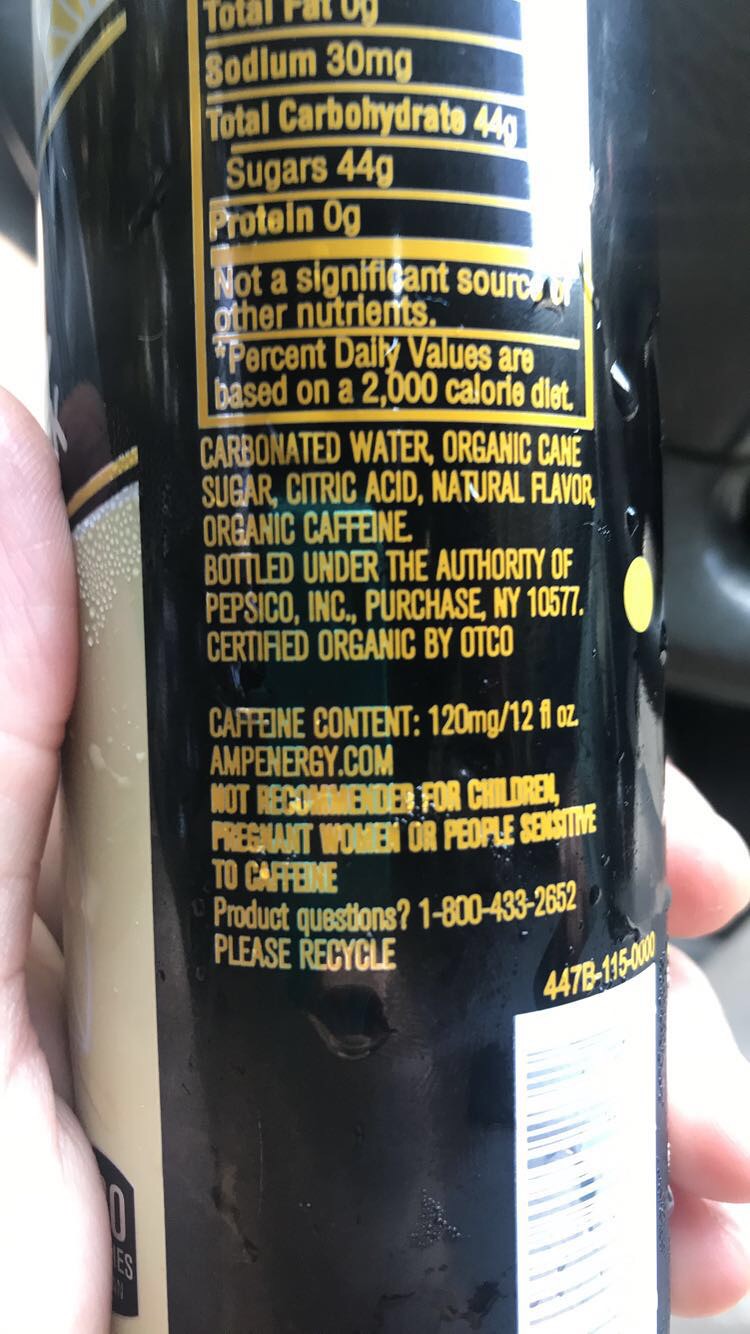This color photograph captures a close-up view of a black, tall, and slender can, believed to be an energy drink, held by a hand against a smartphone. The golden-yellow font on the can stands out with its nutritional information and ingredients. Notably, the top and bottom edges of the can are cropped out of the image. The visible details include a caffeine content of 120 milligrams per 12 fluid ounces and a sugar content listing 44 grams of carbohydrates. Key ingredients such as carbonated water, organic cane sugar, citric acid, natural flavor, and organic caffeine are clearly listed. The label also indicates it is bottled under the authority of PepsiCo Inc., New York, 10577, and prominently displays the URL AmpEnergy.com. Additional details include directives to recycle and a partially visible UPC code with visible black lines against a white background. The product is not recommended for children, pregnant women, or individuals sensitive to caffeine.